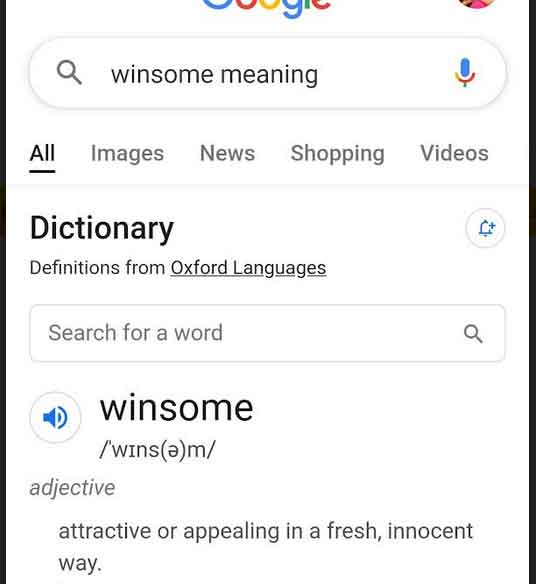At the top of the image, viewers can see the lower portion of the iconic Google logo, featuring its trademark colors: blue, red, yellow, blue, green, and red. Below this, within a search bar, there's a magnifying glass icon on the left and a speaker icon on the right. The search query displayed next to the magnifying glass reads "Winsome Meaning." Directly beneath the search bar, a menu with options like "All," "Images," "News," "Shopping," and "Videos" is visible.

Further down, black text reads "Dictionary," followed by "Definitions from Oxford Languages," both underlined. Below this, there is another bar resembling a search box with the prompt text "Search for a word." A circular blue speaker icon appears next to the word "winsome," spelled out in capital letters as "W-I-N-S-O-M-E." Underneath, the text indicates that "winsome" is an adjective and provides the definition: "attractive or appealing in a fresh, innocent way." This section effectively gives the definition of the word "winsome."